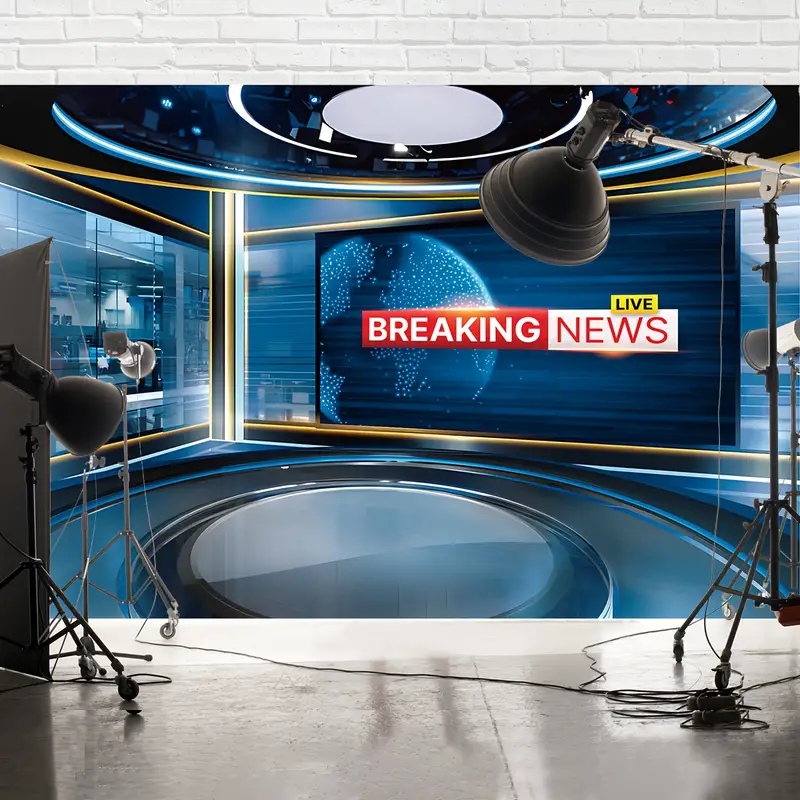This detailed photograph, taken indoors, showcases a modern newsroom studio. The image is square, approximately five inches by five inches, and features a white-painted brick wall at the top half inch of its upper left and right corners. Below the brick section, the studio reveals a higher platform with a gray cement floor located at the lower edges of the photo.

Central to the image is a stage setup accentuated by prominent blue tones—the walls, ceiling, and flooring are a striking blue hue. The main studio area includes numerous tall studio lights aimed at a circular platform in the center, which is devoid of furniture. Overhead, circular lights illuminate this central platform, adding to the professional ambiance.

On the right-hand side backdrop of the stage, there's a significant rectangular banner. The banner reads "Breaking News," with "Breaking" in white print against a red background on the left, and "News" in red print against a white background on the right. Above this banner is a smaller yellow rectangle with "Live" written in black text, signifying live broadcasting status. The digital screen backdrop also features an illustration of Earth in dark and light blue, with white dots highlighting various locations.

The studio's floor is cluttered with numerous black electrical and microphone cords snaking around. There's also a mention of some office equipment visible through what appears to be a glass window wall, adding depth to the studio setting. Additionally, gray cloth structures and mobile grey headlamps on wheeled stands are also seen, further ensuring optimal lighting for the studio.

The image encapsulates a bustling, well-equipped news studio ready for broadcasting.